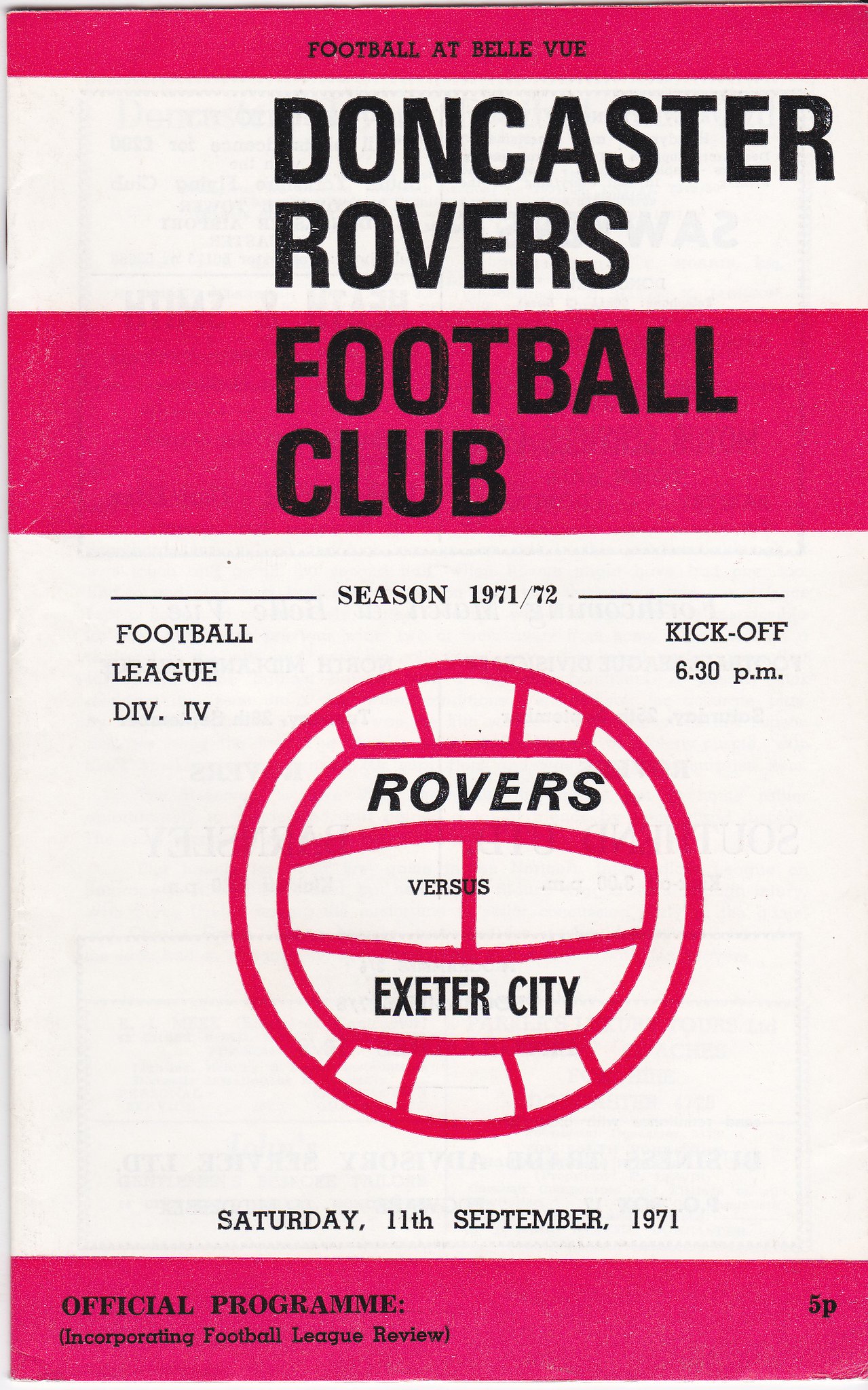The cover of the official program for the Doncaster Rovers Football Club, specifically for the match between Rovers and Exeter City on Saturday, the 11th of September, 1971. The design features a prominent red bar at the top with the text "Football at Bellevue" in black. Below that, "Doncaster Rovers" is boldly printed in black on a white background, followed by another red bar containing "Football Club" in black letters. Central to the cover is an intricate soccer ball illustration with red stripes, inside of which "Rovers vs. Exeter City" is written in black letters. Alongside the soccer ball, on the left, "Football League Division IV" in Roman numerals and "Season 1971-72" are inscribed, while on the right, "Kickoff 6.30 p.m." is noted. At the bottom, another red horizontal bar contains "Official Program" in black, alongside the price of five pence. Beneath this, in smaller print, the cover states, "Incorporating Football League Review". The overall color scheme features white paper with red and black elements, creating a striking, tri-chrome aesthetic.